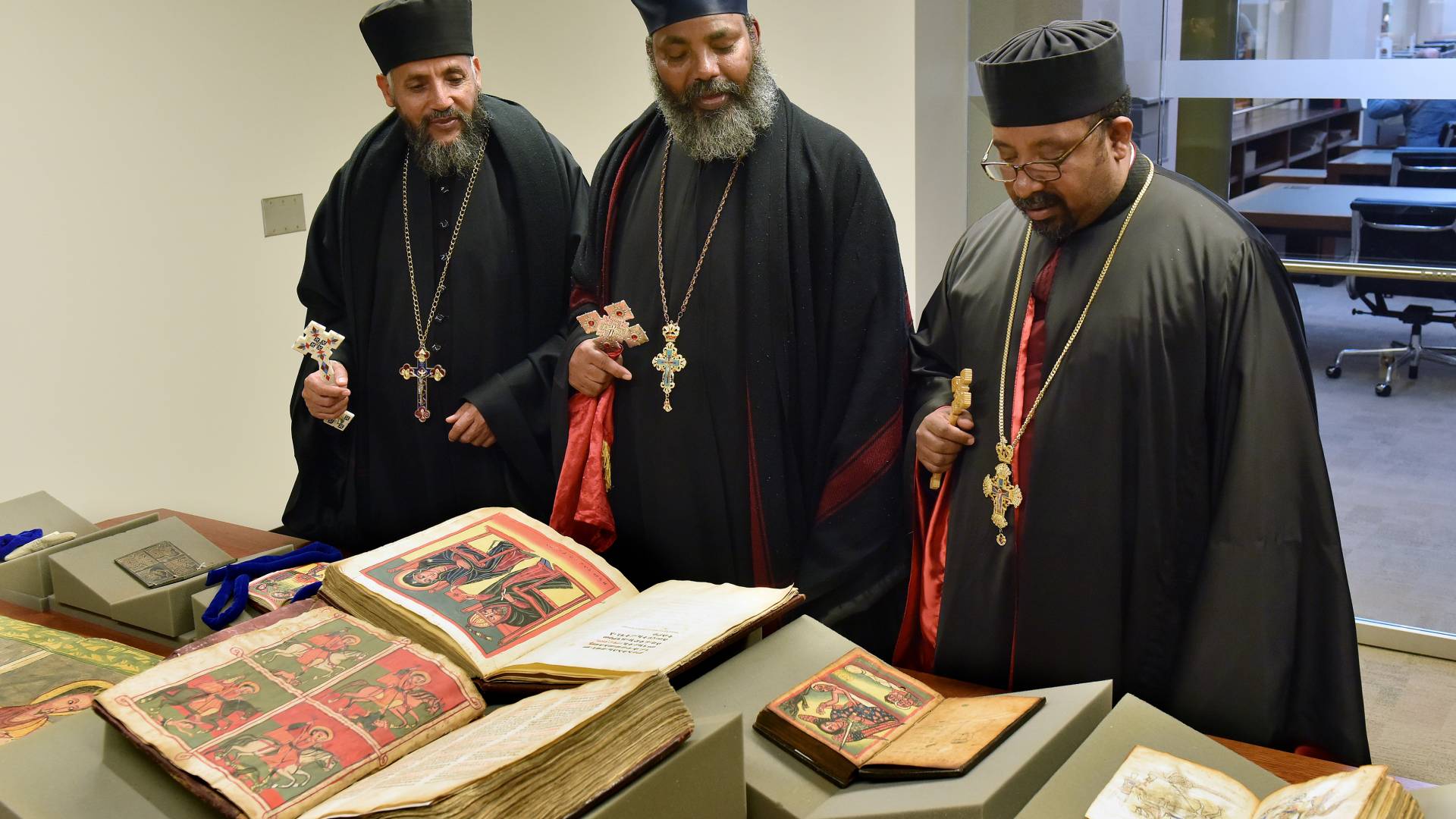The indoor photograph captures three African-American clergymen, likely Eastern Orthodox or Russian Orthodox priests, standing in a room that looks like a hybrid between an office and a museum. They are dressed in long black robes with hints of red on the inside, and each wears a round black hat. Gold necklaces with crucifix medallions hang around their necks, while they hold intricately detailed crosses in their right hands. All three men have beards, and the one on the far right wears glasses. They are intently reading from a selection of open scripture books that feature illustrated Christian imagery, with some pages appearing old and yellowed. The table in front of them holds about four or five of these ancient-looking books. In the background, a tan wall is visible on the left, and a glass wall on the right reveals an office setting with desks and chairs. The men, appearing to be in their mid-40s to early 50s, are deeply engrossed in their reading, contributing to the solemn and reverent atmosphere of the scene.